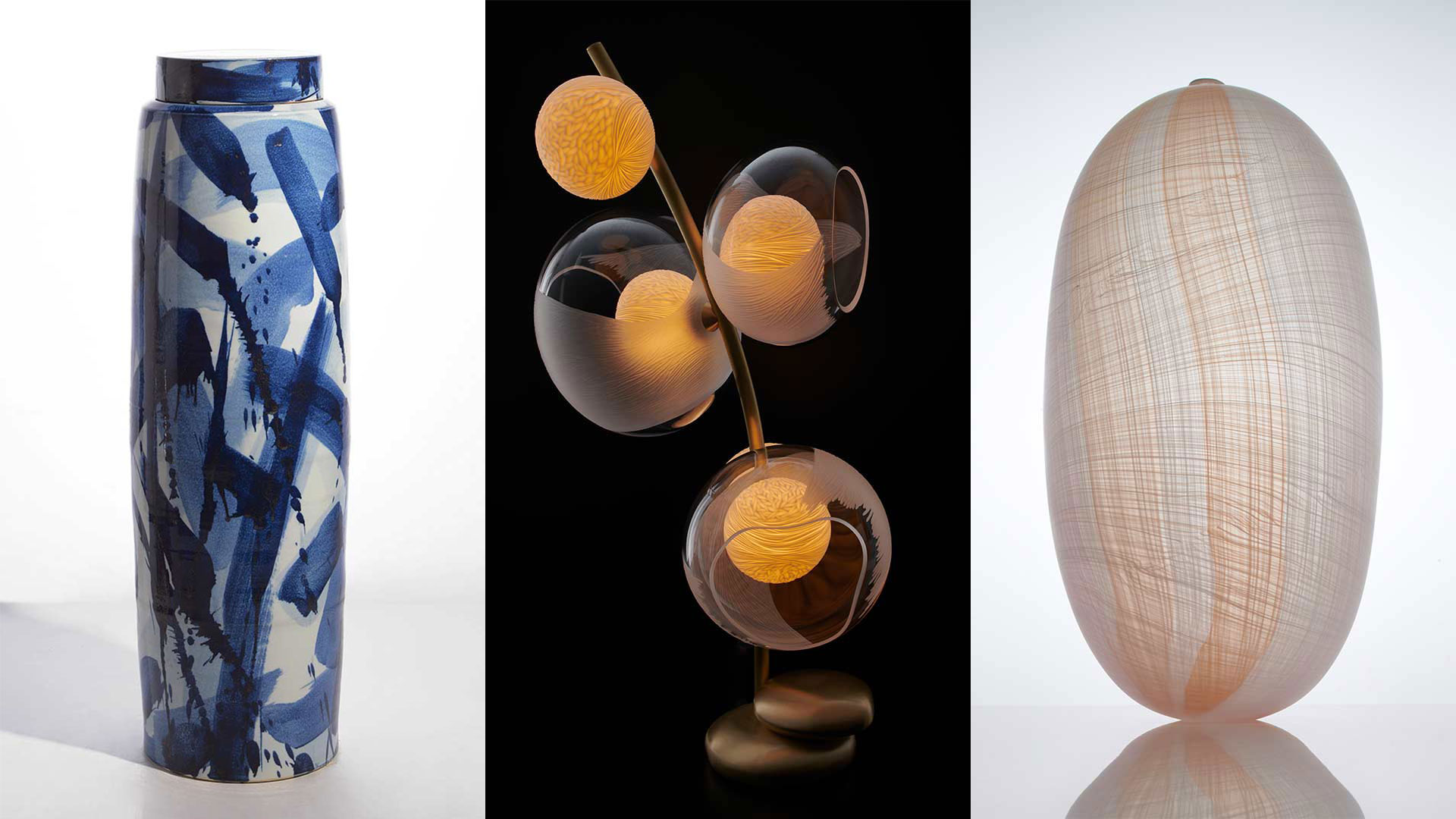This image consists of three distinct objects, each showcased in separate photos aligned in a row. The leftmost photo features a tall, slender canister with a blue lid. The canister is artistically painted with various shades of blue, white, and black patterns, creating an intricate design. The central image displays a uniquely designed lamp or lighting sculpture. This piece has a black background and is characterized by a metal rod suspending a series of illuminated orbs. These orbs appear to be made of glass, each containing a smaller glowing nucleus, and are arranged in a circular pattern around the rod. The setup includes a brown base and a combination of glowing yellow and clear elements. Finally, the rightmost photo presents an oval-shaped glass sculpture with a balloon-like appearance, set against a white background. The sculpture boasts a crosshatched design featuring orange and gray hues, with a reflective surface that enhances its wavy, blown-glass aesthetic.